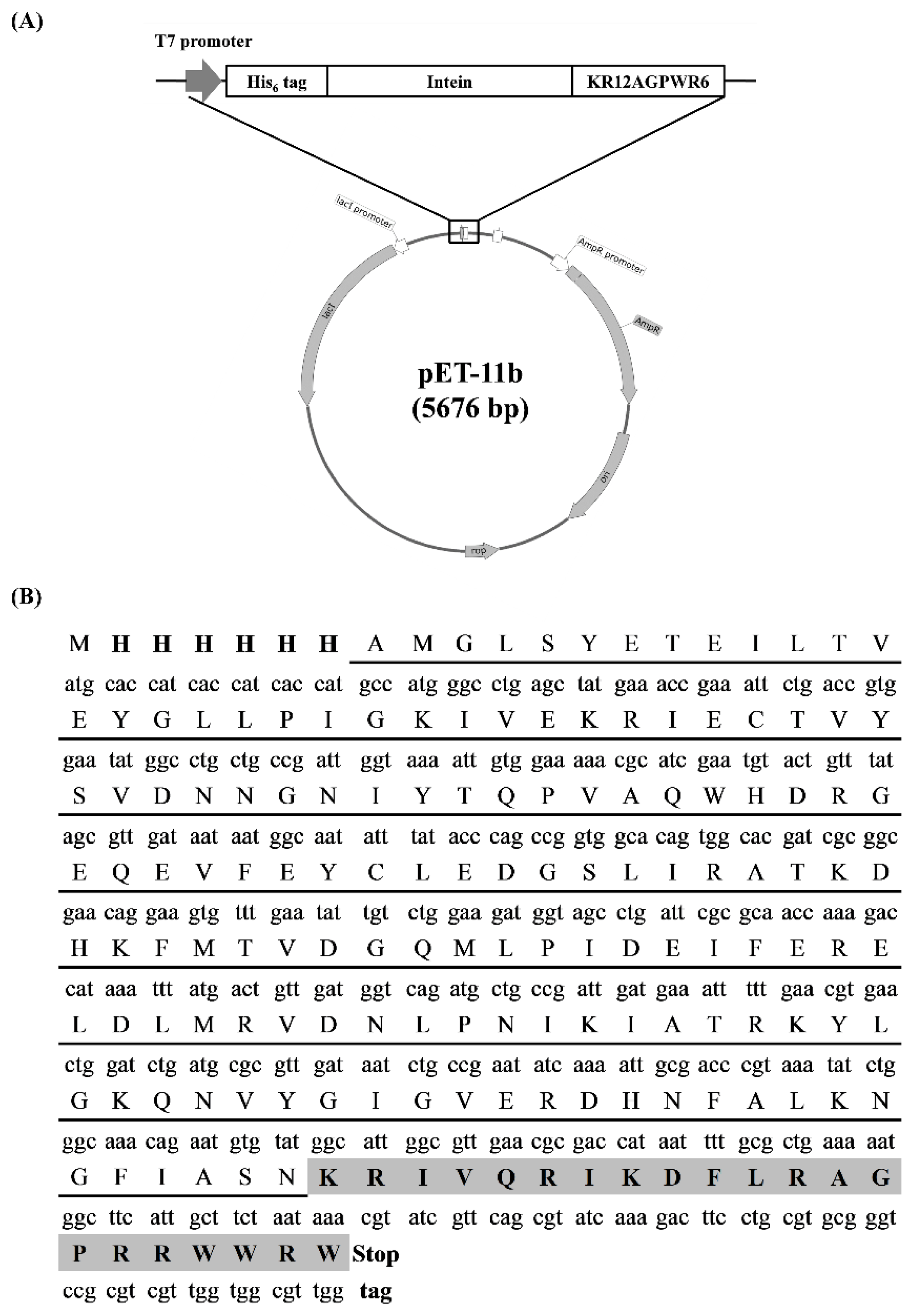The chart displays a sequence of letters and numbers that appear to be part of a scientific analysis or dataset. At the top of the chart, there is a gray circle labeled "PET-1111B (5676PB)" with an adjacent "B" designation. The rows beneath this header contain repetitive sequences of letters. The first row starts with "M H H H H H H" followed by "A T G | C A C | C A T | C A C | C A T | C A C | C A T" and then continues with "M G A | M G." This pattern is likely representative of a specific type of scientific or molecular sequence, though its exact significance is not clear.